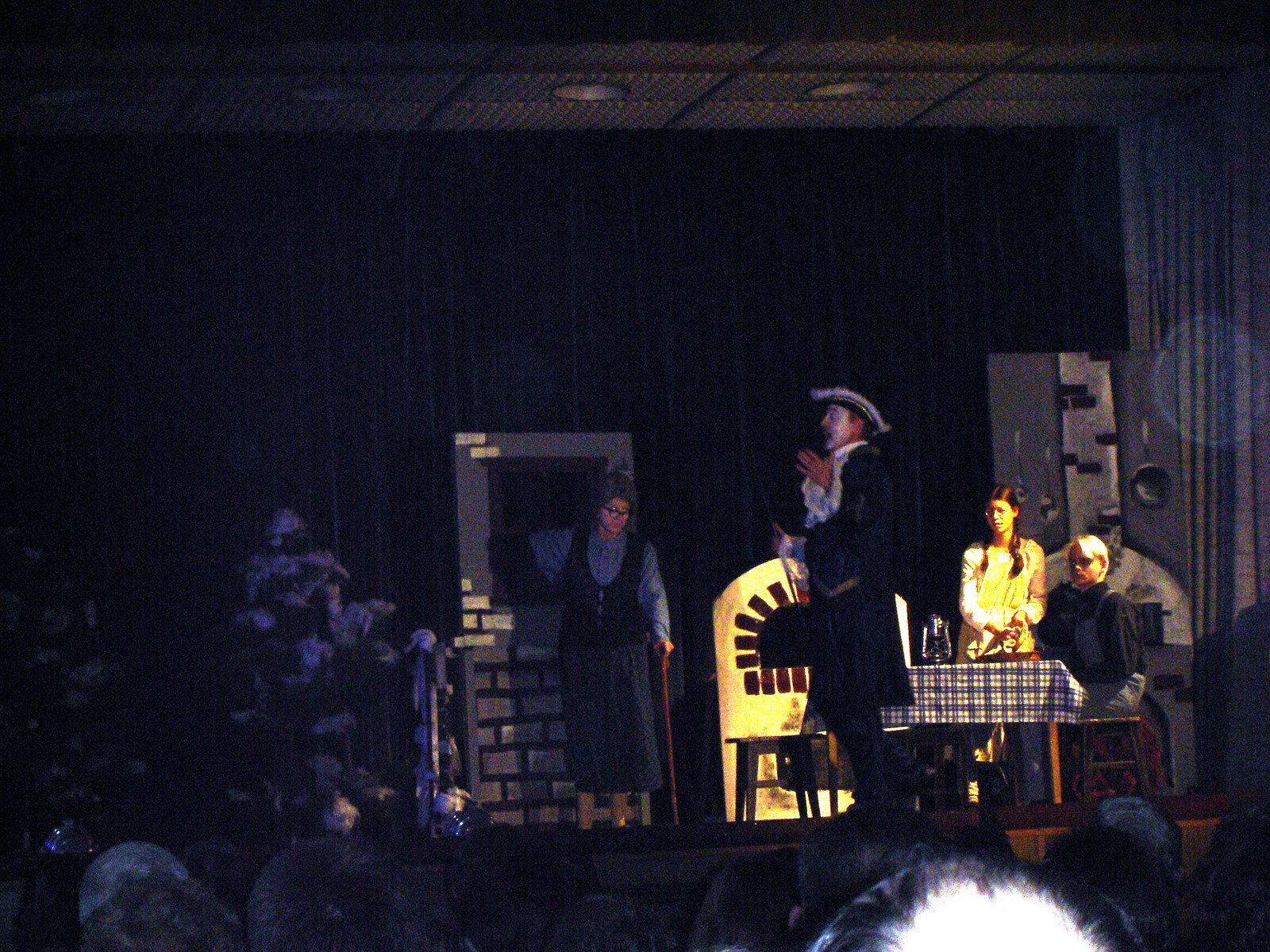This image captures a moment from a theatrical performance set in a dimly-lit theater, emphasizing the dramatic atmosphere of a night scene. The stage is dark, illuminated primarily by a single bright yellow light on the right-hand side, which highlights the actors' faces. The backdrop is a black curtain that adds to the subdued lighting. The focus of the scene is a passionately speaking man, distinguished by white face paint, wearing a costume reminiscent of a British colonial soldier in blue attire with a tricorn hat. He paces across the stage, hands raised expressively.

To the right of the image, seated at a table covered with a blue checkered tablecloth, are two children—a boy and a girl—looking intently at the man. On the left, an elderly woman dressed in a black vest over a light blue button-down shirt and a long gray skirt stands against a gray prop wall. She leans on a cane, with gray hair and glasses adding to her historical look. The scene is part of an evocative historical reenactment, with the audience's heads faintly visible at the bottom of the picture, engrossed in the unfolding drama.